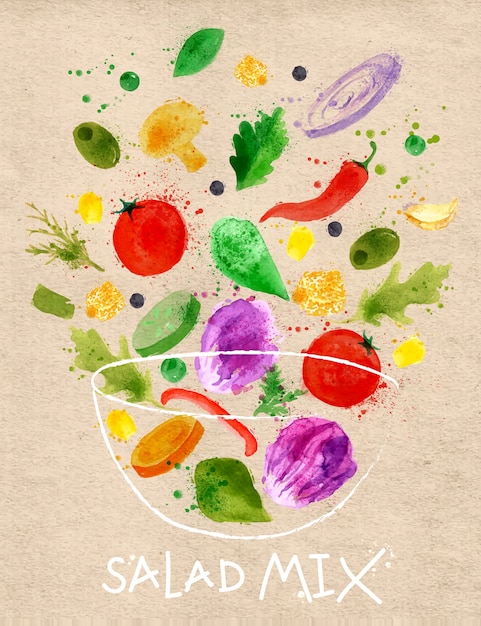This is a detailed illustration titled "Salad Mix," set against a cream-textured or light gray background. The composition features an assortment of vibrant vegetables artfully arranged, appearing to float both within and above a transparent, white-outlined bowl. Prominently featured are red onions, peppers (both bell and chili), olives, various lettuces, mushrooms, tomatoes, and radicchio, along with elements like peas, cabbage, and herbs. Some vegetables are depicted whole, such as the tomatoes and peppers, while others are shown sliced, offering a loose, abstract representation. The colorful ingredients are evenly spaced yet arranged in a dynamic way, creating an impression of them almost flying out of the bowl. At the bottom of the image, the words "Salad Mix" are written in white, underscoring the playful yet organized chaos of this artistic salad medley.